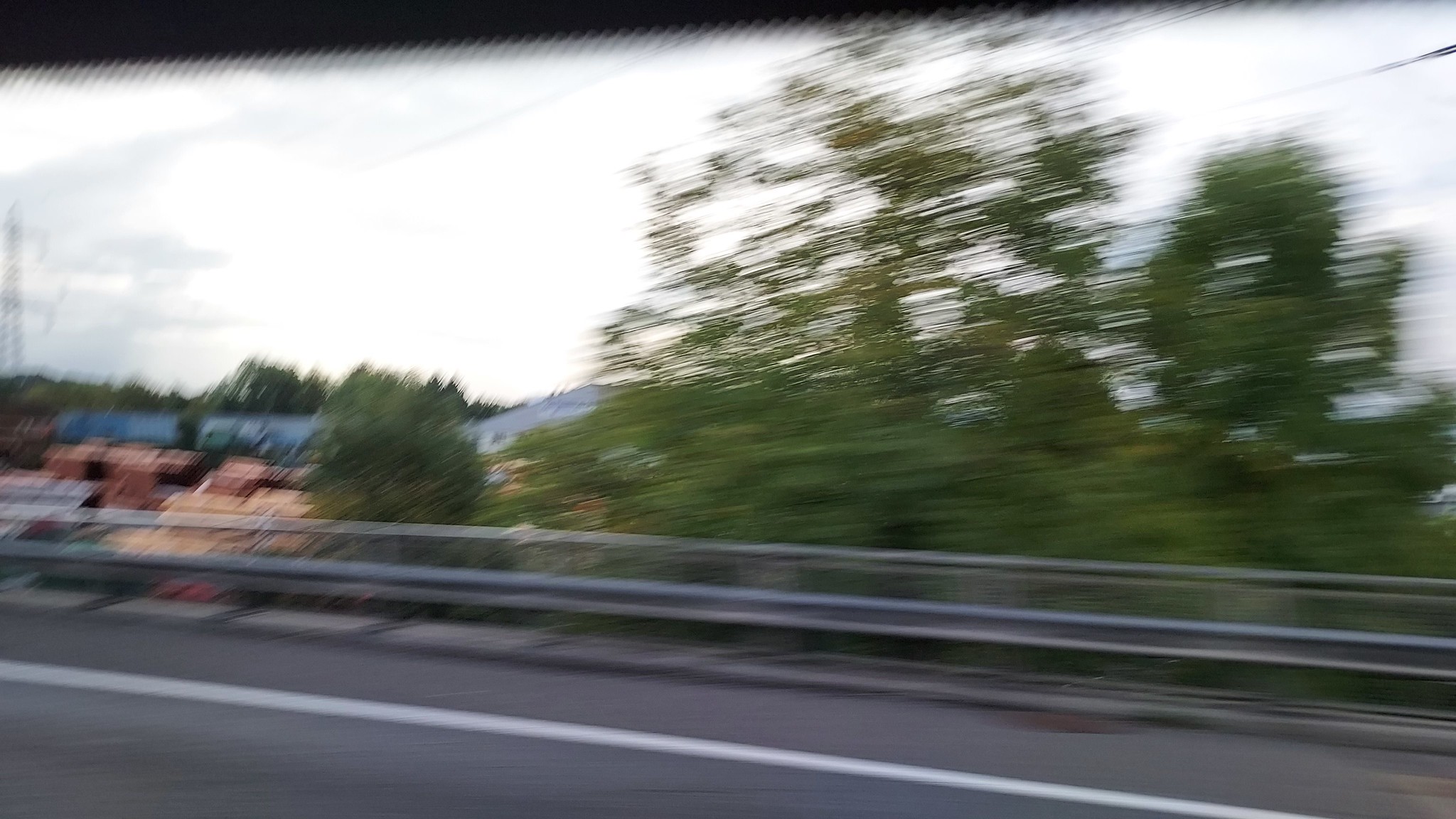This image, taken from a moving car and slightly blurry due to the motion, captures a first-person perspective looking out the side window of a vehicle. In the foreground, the light gray road is visible with a distinct white line marking its edge. Adjacent to the road is a metallic, rectangular fence-like barrier, designed to prevent vehicles from going off the edge, suggesting the road is on a higher elevation, possibly a bridge or a mountainside. Beyond the railing, there is a drop-off leading to an area with tall trees featuring light green leaves, positioned on a lower surface. Towards the left center of the image, some residential buildings are visible, showcasing a mix of beige, red, and white colors. Further in the distance, a small blue lake surrounded by additional trees can be seen. The sky above is dull and overcast, adding to the overall muted tone of the photograph. Part of the car's window frame is visible at the top of the image, indicating the photograph was taken from inside the moving vehicle. No people, animals, or other vehicles are present in the shot.